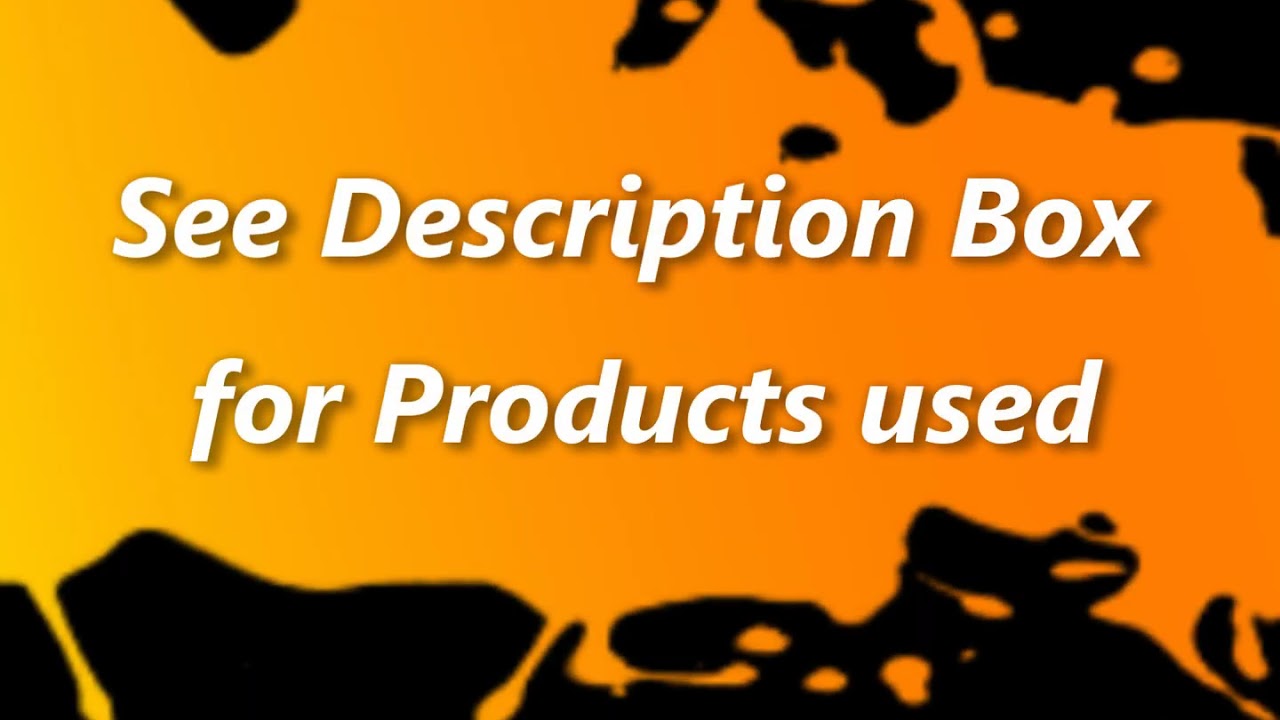The image is a horizontal graphic with a yellow-to-orange gradient background, resembling a paint splatter effect that transitions from yellow on the left to orange on the right. The splatter, which covers the middle portion of the graphic, has black ink blotches and blobs around the borders, extending slightly inward. Some of these black splotches appear on the sides and bottom, with a few resembling claw-like shapes. Centered in the middle of the image, two lines of white text with a slight drop shadow read, "See description box for products used." The layout is longer left to right than it is top to bottom, with the black shapes providing a striking contrast against the vibrant background.